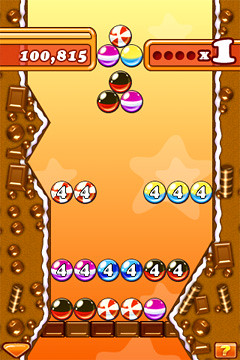This image is a screenshot of a very old, decades-old video game featuring simple, non-photorealistic graphics. The screen is divided into various sections with a prominent vertical rectangle in the middle. The background features an orange gradient transitioning from a deep orange at the bottom to a light yellow at the top, embellished with pale gray stars. On the right and left sides, there are brown areas that resemble chocolate, each taking up about 10% of the screen with a white outline along the edges.

At the top of the screen, a bold score is displayed in bright orange with white text reading "100,815." To the right of this score is an indicator for Player 1 denoted by "X1." The primary focus is on the colorful marbles scattered across the screen, arranged in various patterns. These marbles come in colors such as red, purple, white, black, blue, and yellow, with some in the middle displaying numbers in white.

At the bottom, a row of square chocolate pieces forms a border, containing an array of circular marbles. In this section, six marbles of different colors like aqua blue, orange, and maroon are aligned side-by-side. Ascending towards the middle, there is a row of numbered marbles, while higher up, clusters of marbles are arranged in triangular formations.